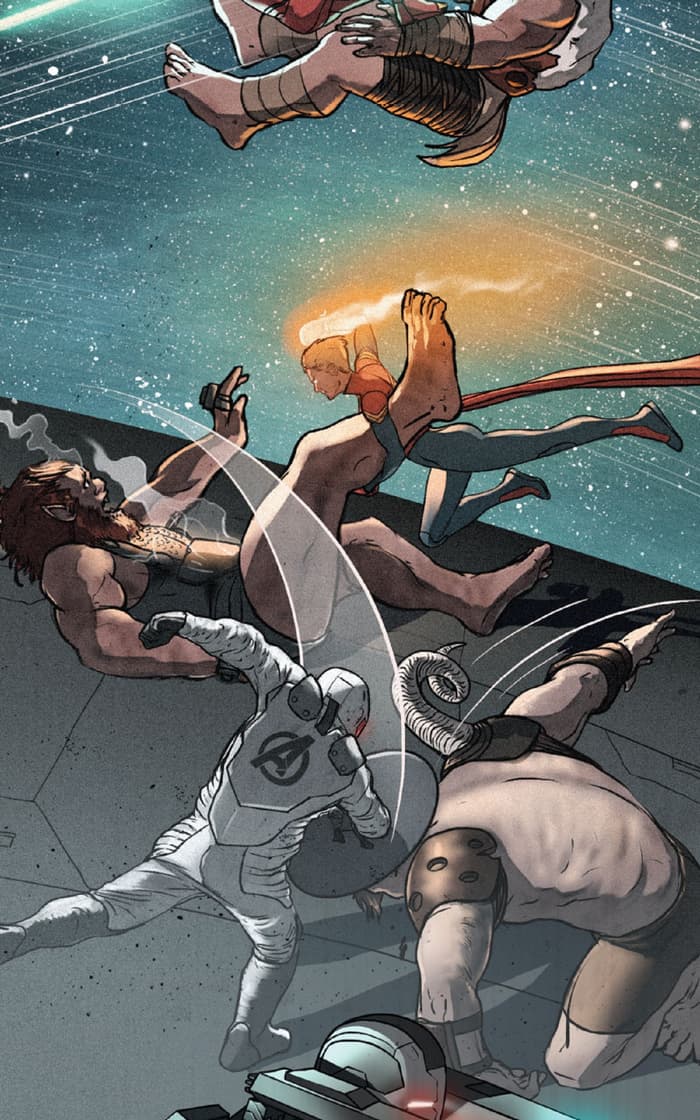The image is a vertically aligned, borderless comic strip depicting an intense battle scene inside a spaceship. The background through a large window reveals a starry expanse of blue and gray filled with tiny white spots representing stars. At the very top of the image, partially visible, a person's foot, leg, and part of their hand float into the scene. 

In the upper center, a man with blonde hair in tight gray pants and an orange shirt is flying through the air, emanating flames from his hand towards a kneeling giant. This flame-throwing action suggests a fierce attack on the giant below. On the lower part of the image, a figure in a gray-silver full-body suit with an "A" logo within a circle on its back is wielding a large silver shield. He appears to be striking a beast or monster with fangs on the head in a swooping motion. The ground beneath them is made up of large geometric gray shapes. 

Lying in the middle of the foreground is a muscular man with abundant brown hair and facial hair, reaching up, possibly in a defensive or pleading gesture. The scene is chaotic and highly dynamic, emphasizing action and conflict among the characters in what appears to be a technologically advanced, interstellar setting.